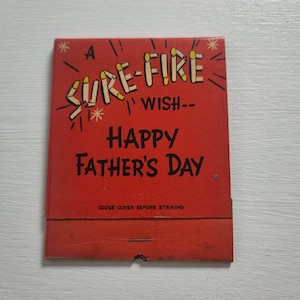The image showcases a vintage red matchbook lying on a light wood table with a soft gray or white background. The matchbook appears old, possibly over 20 years, but is in good condition. The front cover of the matchbook features the phrase "A Surefire Wish, Happy Father's Day" in all caps. The word "Surefire" stands out as it is creatively depicted using matchsticks with yellow tips, resembling fireworks or matches ready to ignite. Below this, in small black font, the instructions "Close cover before striking" are visible, along with a staple securing the paper together over the matches. The overall presentation is simple, with no other significant elements in the photo.